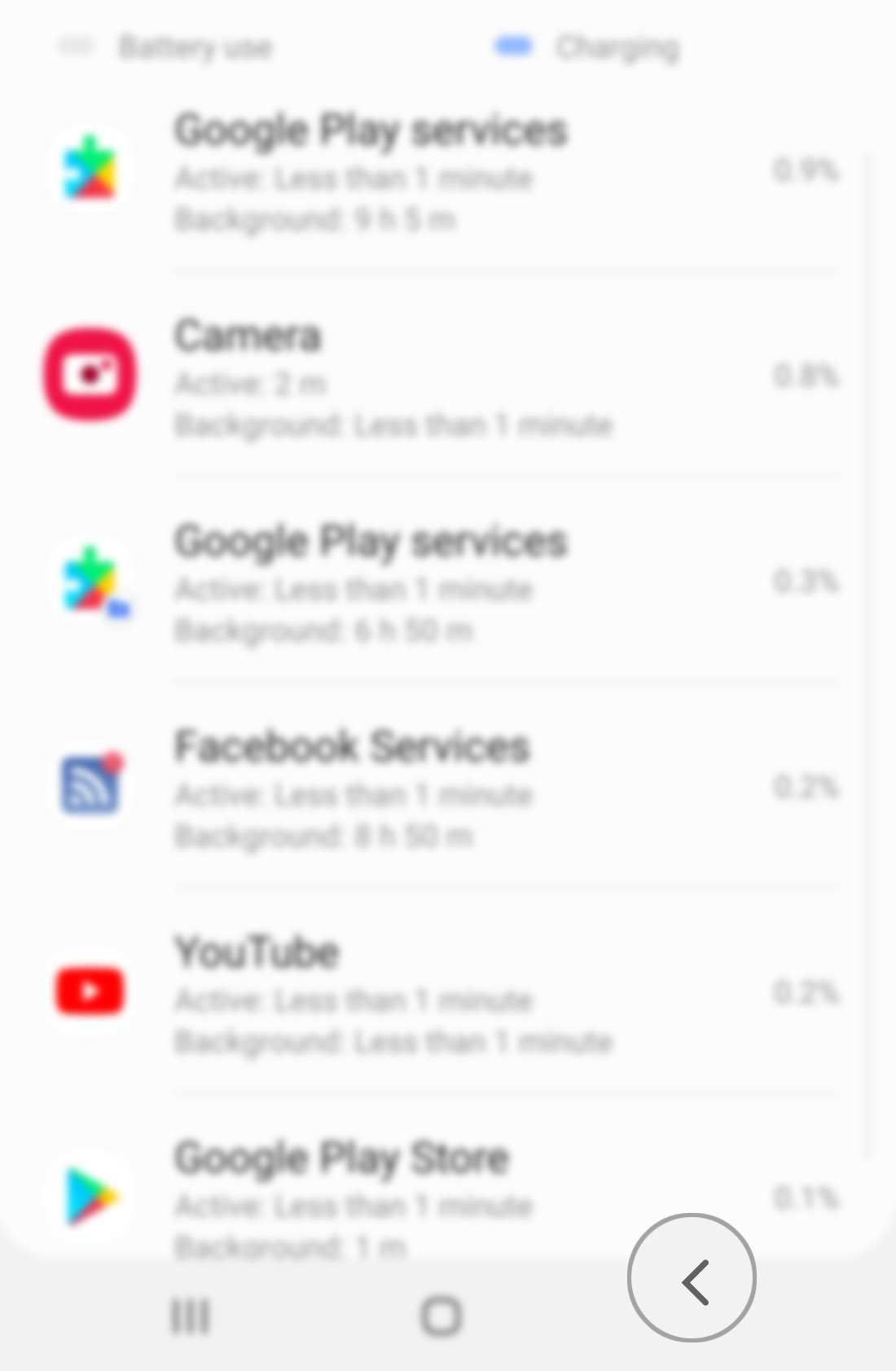A very blurry image shows a smartphone screen with an out-of-focus menu. At the top of the screen, the battery icon and charging status are visible. Below it, a section appears to list various services and applications along with their respective battery usage percentages. The readable entries include Google Play services, the camera, more Google Play services, Facebook services, YouTube, and the Google Play Store, each accompanied by a percentage value. The larger text is discernible, but smaller font details are illegible. The background features a mix of blue, green, yellow, red, white, dark blue, lighter blue, and gray colors. Navigation icons are present at the bottom, including a gray and white outlined circle with a left arrow. The overall impression suggests the screen is displaying battery usage details while charging, with Google Play services consuming 0.9%, the camera 3%, and another instance of Google Play services also taking 3%. The image is significantly out of focus, making it challenging to identify finer details.